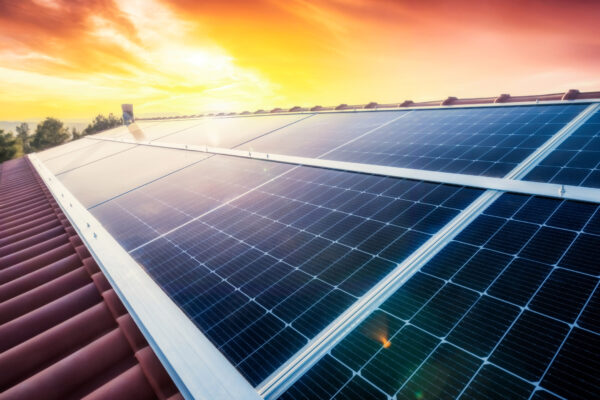This photograph captures a rooftop adorned with an extensive array of large solar panels. The panels are arranged in two rows, seamlessly covering almost the entire visible section of the roof, with twelve panels clearly discernible. Each panel is composed of numerous small black rectangles divided by thin white lines, all enclosed within white frames that subtly reflect the colorful sky. The roof itself, featuring reddish-brown shingles with a rounded design, comes to a peak, adding a dynamic structure to the scene. Below the roof's edge, trees peek out, adding a touch of nature to the image. The backdrop is a stunning sunset, with a sky ablaze in hues of gold, yellow, pink, bright reds, and deep reds intermingling with scattered clouds, creating a spectacular and serene atmosphere.